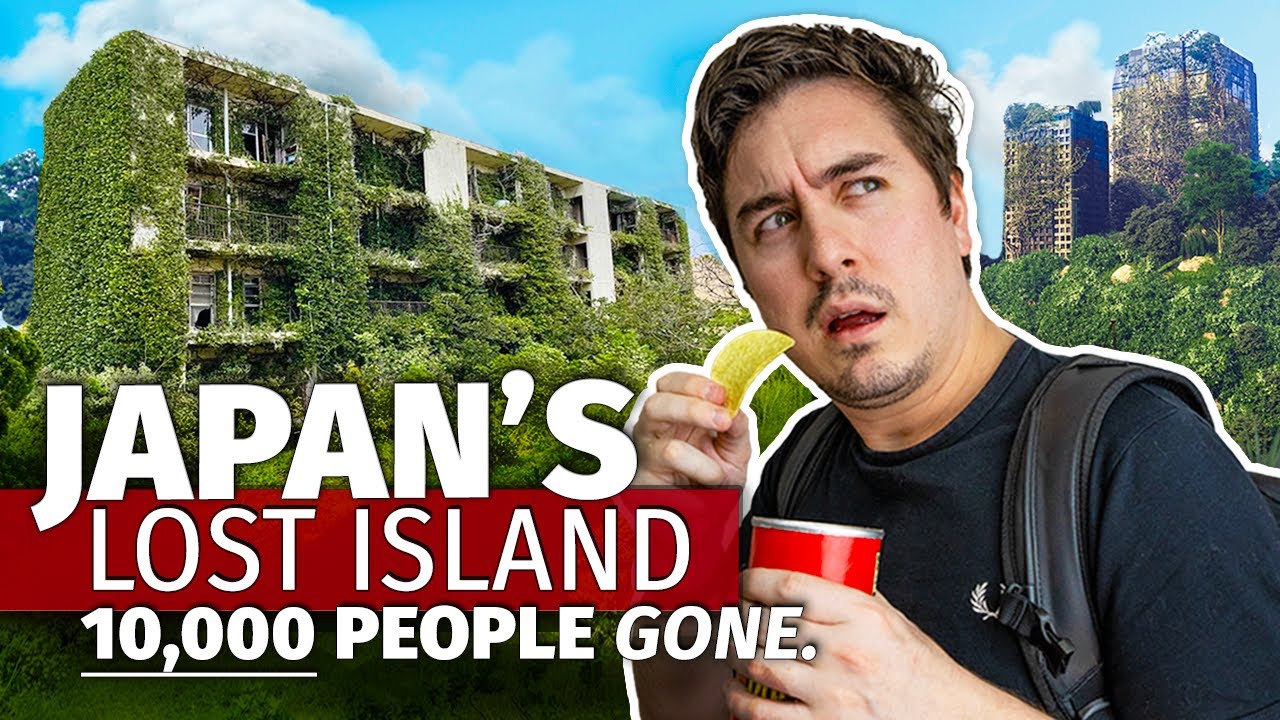The image depicts an overgrown cityscape with high-rise structures enveloped in dense green ivy and vegetation, indicating abandonment. The foreground showcases a man, likely American, with short brown hair, blue eyes, and a bit of stubble, wearing a black short-sleeved T-shirt and a backpack. He appears confused, looking up to the upper right while eating a Pringle and holding a red Pringles can. The sky above is light blue with scattered white clouds. Overlaying the image, bold white text reads, "Japan's Lost Island, 10,000 People Gone," with "Lost Island" highlighted by a red border and "gone" italicized, suggesting a mysterious or dramatic context, perhaps for a YouTube thumbnail.